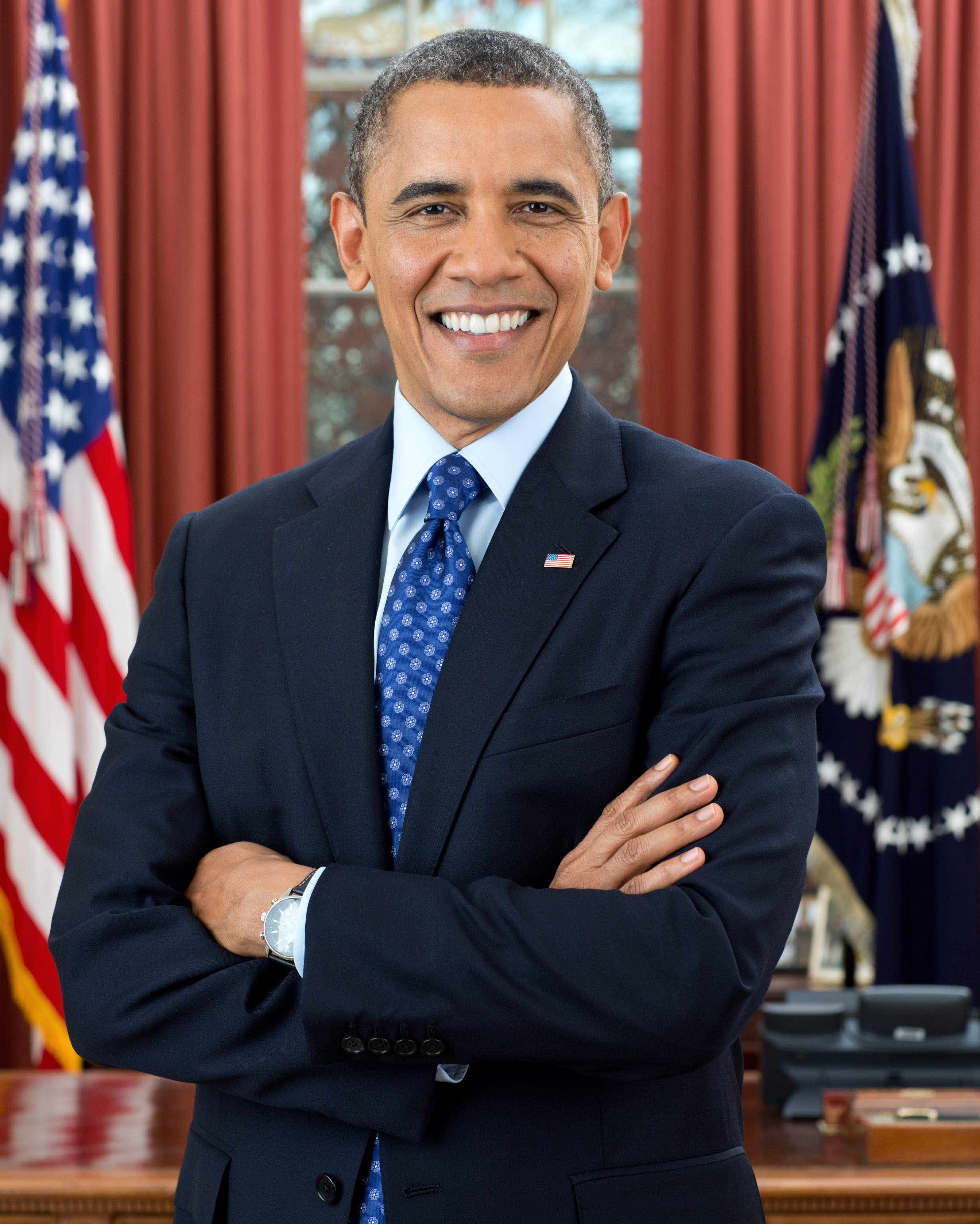This is a detailed photograph of United States President Barack Obama, taken during his tenure in the Oval Office at the White House. President Obama is positioned in front of a desk with his arms crossed, exuding a sense of happiness and relaxation as he smiles broadly. He is dressed in a dark navy blue suit paired with a white button-down shirt and a blue tie that features a subtle white pattern. Adorning his left lapel is an American flag pin. Obama, a medium light-skinned male of African and Caucasian descent, stands confidently in front of the iconic setting.

In the background, a large window typical of the Oval Office is framed by elegant red draped curtains. To the left of the desk, the American flag is prominently displayed, while to the right, there is a blue flag featuring an eagle holding arrows, likely representing the Presidential seal. The overall composition of the photograph, with its rich details of attire, setting, and symbolism, captures a moment of presidential dignity and warmth, reflecting both the man and the office he holds.